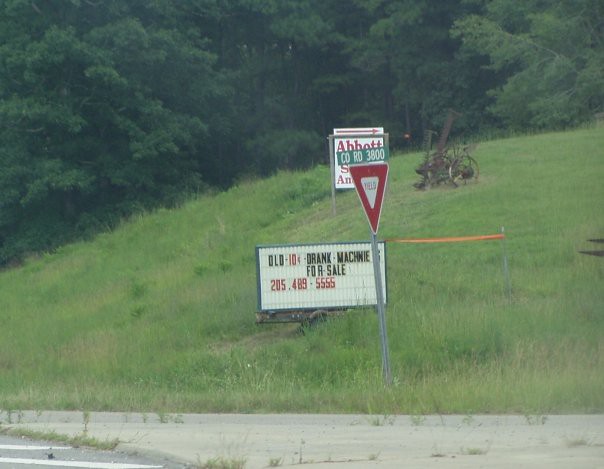This photograph appears to be taken from a moving car, capturing a hill in a grassy area with thick, dense trees in the distant background. At the top of the hill, there's an old-fashioned farm tiller that is bronze or rust-colored. Near the base of the hill is a trailer with two wheels, featuring a white letter sign commonly used for advertisements. The sign, with black and red letters, reads "Old 10 cent drink machine for sale" and lists a phone number, 205-489-5555, in red letters. Adjacent to the trailer, there is a yield sign, partially obscured by a green street sign indicating "County Road 3800." Further in the background, another sign is visible, which reads "Abbott" with an arrow pointing, though it is also partially blocked by the yield sign. The road is visible at the bottom of the photo, with grass either growing or scattered across it.